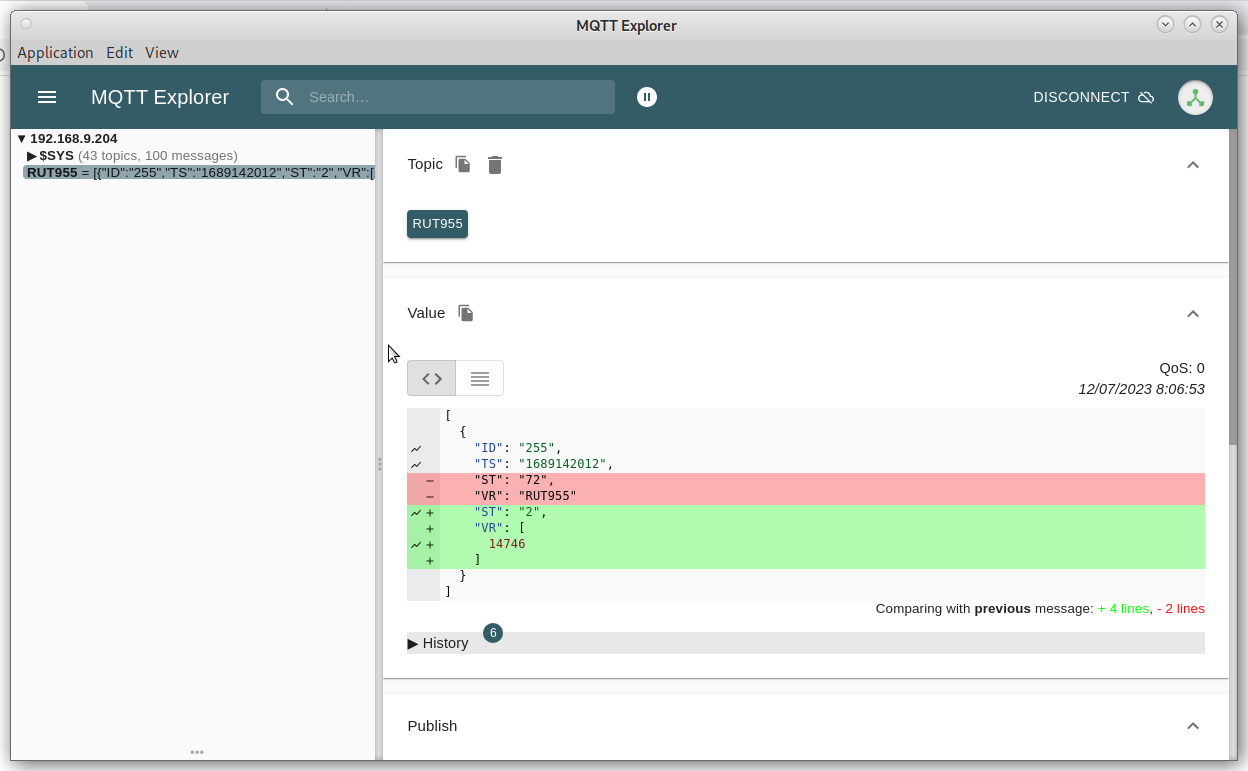The screenshot depicts the user interface of an application named "MQTT Explorer," a web-based tool for exploring and debugging MQTT connections. The layout features a classic menu bar at the top with three primary menus: "Application," "Edit," and "View." Below this menu bar, a dark green navigation strip runs horizontally across the screen, displaying white text. On the far left of this strip is a clickable three-bar menu icon, often referred to as a "hamburger" menu. Next to this icon, "MQTT Explorer" is displayed prominently.

Situated to the right of the "MQTT Explorer" text is a search bar containing a microscope icon and the word "Search." Farther to the right, the word "Disconnect" is paired with a cloud icon struck through with a line, signifying a disconnection option. Adjacent to this, another icon displays three dots connected by lines, likely indicating additional settings or a network map.

Beneath these options, a detailed panel shows the IP address "192.168.9.204," accompanied by a sub-menu. Initially, it reveals metrics stating "43 topics" and "100 messages." To the right of these statistics, three bars in white, pink, and green are displayed, each labeled with two-letter abbreviations followed by numerical values. At the bottom of the screen, an option to access history is available, likely providing a log or timeline of MQTT activities.

In summary, this image encapsulates the comprehensive and user-friendly interface of "MQTT Explorer," highlighting key functionalities and connection details for effective MQTT management and debugging.